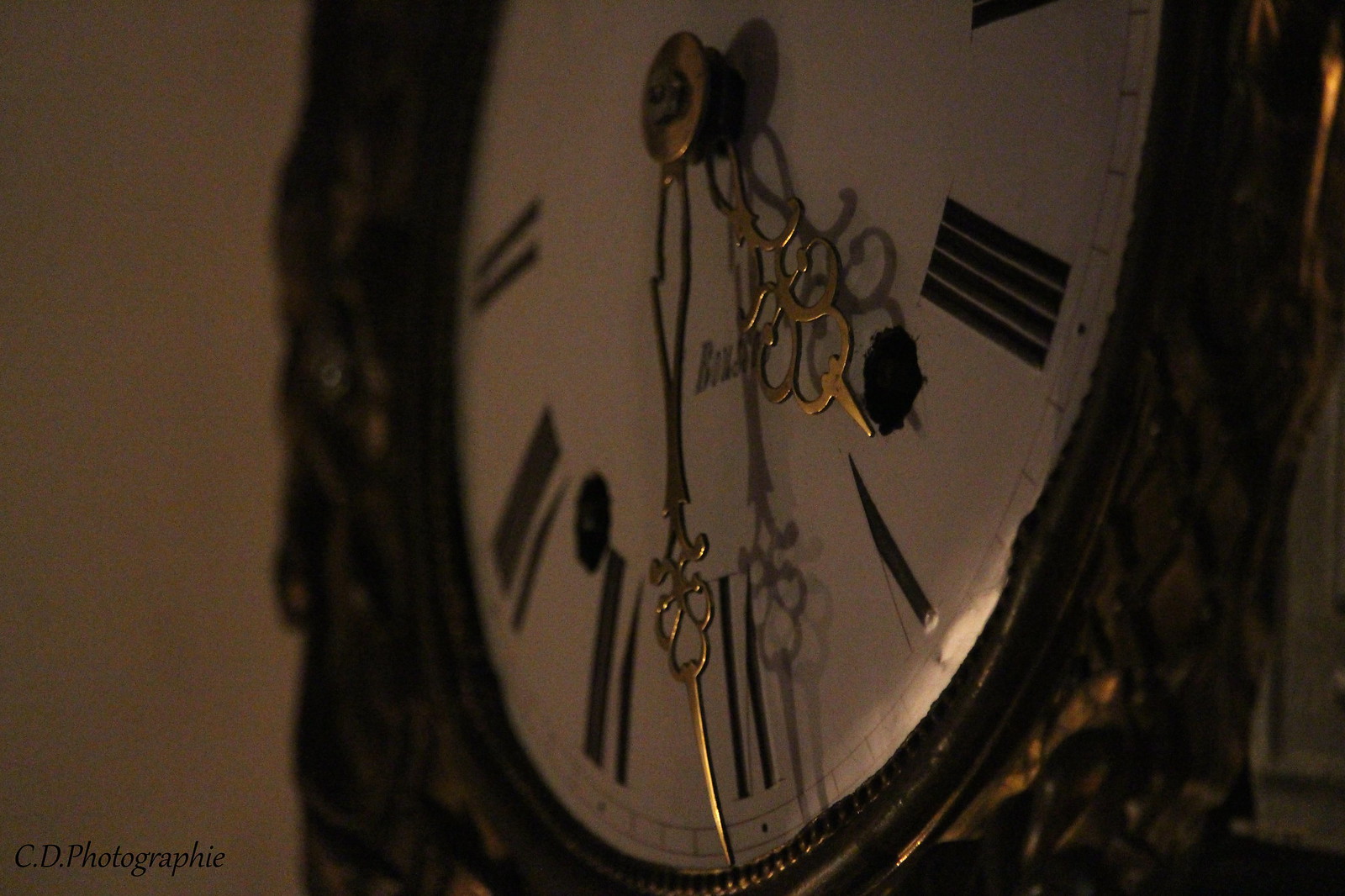The photograph captures a close-up, dimly lit image of an antique or vintage clock, emphasizing its intricate details. The clock's housing appears to be made of brass or a gold-like metal, lending it an aged, classic appearance. The face of the clock is white, though only partially visible due to the tight framing of the image, specifically showing the Roman numerals IV through IX. These numerals are black, contrasting vividly against the white background. Notably, the clock hands are ornate, designed with a golden brass finish, and indicate a time of approximately 4:30, with the short hand positioned between IV and V, and the long hand near VI. A peculiar black spot is present at the clock's center, resembling ink, adding an element of mystery. The lower half of the clock face is more visible, with slight blurring towards the left, enhancing the vintage aesthetic. The name "CD Photography" is subtly mentioned, suggesting the photographer's credit.